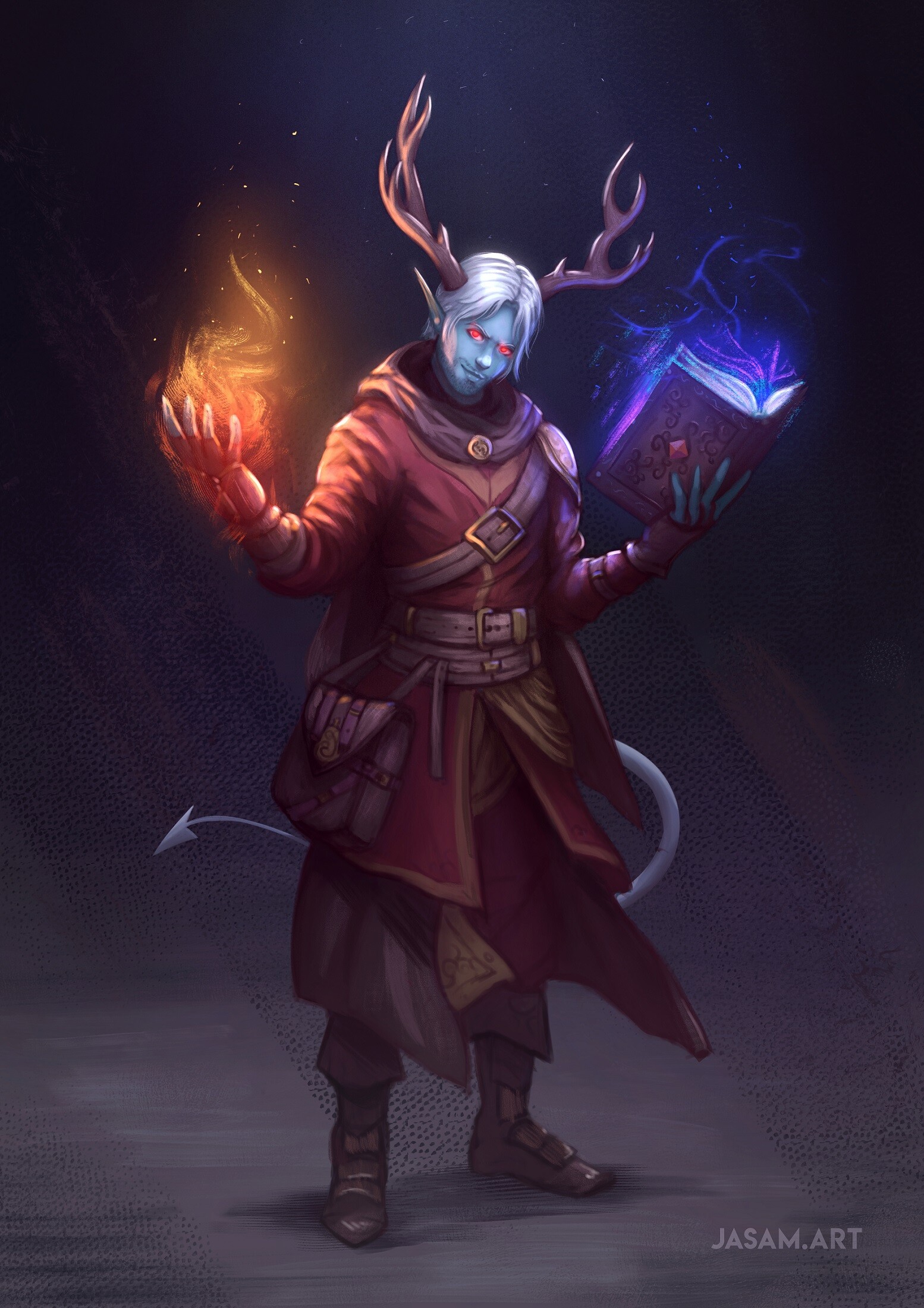The image depicts a demon-like character that evokes a sorcerer or superhero from a comic book or cartoon. Set against a blue-black and purple background with a gray floor, the character stands out with its blue face and long white hair parted at the middle. Dark red eyes add intensity to its youthful appearance, and it sports deer-like antlers protruding from its head. In its right hand, the character holds an open book emitting a blue light, possibly representing spells, while its left hand conjures a ball of flame reaching toward the sky. The demon is dressed in an elaborate brown coat, reminiscent of a soldier or pirate uniform, complete with a cross-chest strap, multiple belts around its waist, and a pouch on its side. A gray tail snakes around the character to the left, adding to its devilish features. Brown boots complete its attire. The artist's signature, "jasm.art," appears in a gray font at the bottom right corner of the image.